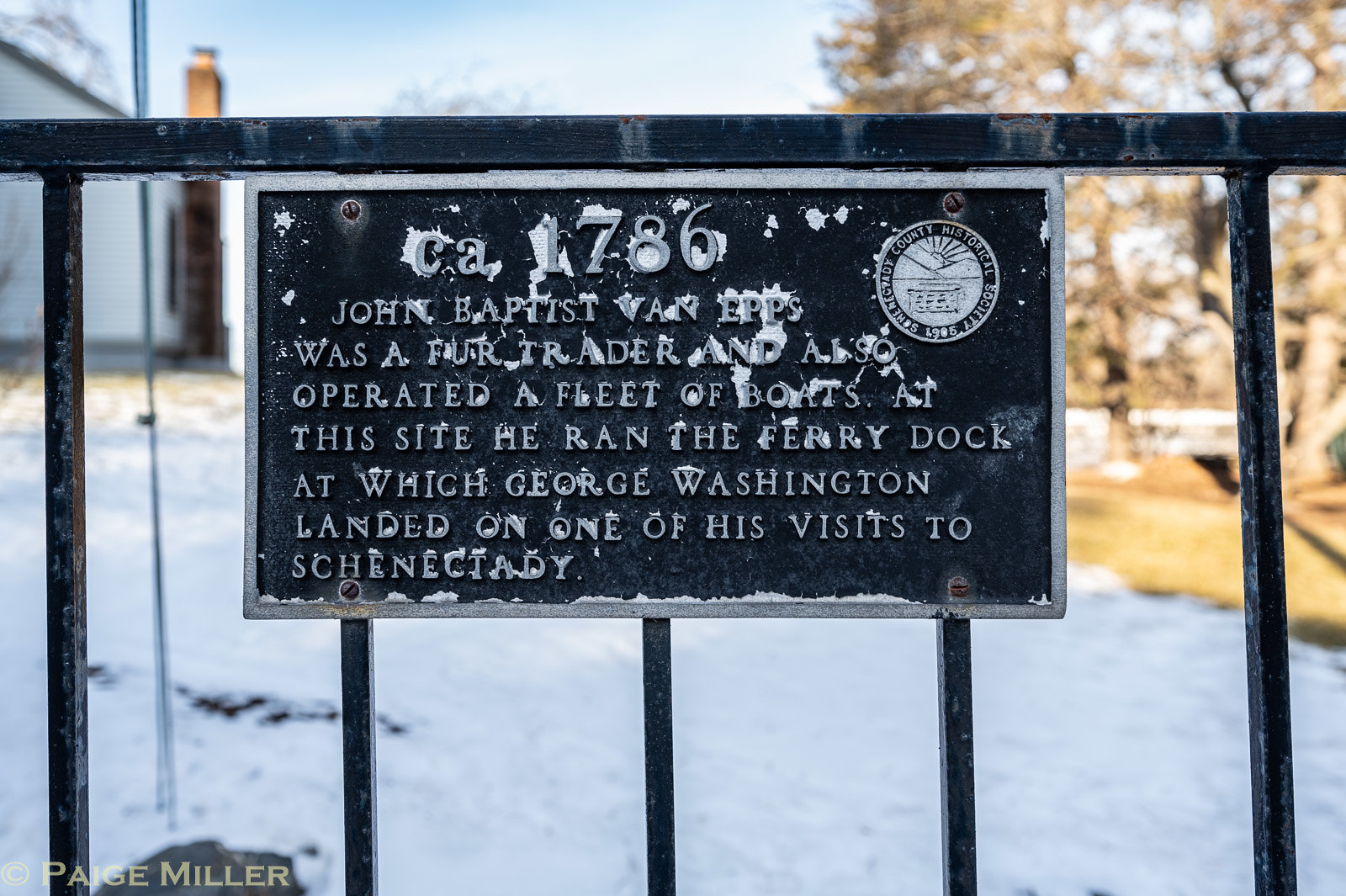In this detailed photograph of a historical marker, we see a black wrought iron gate partially covered in snow, suggesting a winter setting. The background features a house and leafless trees, enhancing the cold, desolate atmosphere. Central to the image is a worn black metal plate, with chipping paint and a silver metal border, securely fastened to the gate. The sign reads, "CA 1786 John Baptist Van Epps was a fur trader and also operated a fleet of boats. At this site, he ran the ferry dock at which George Washington landed on one of his visits to Schenectady." A small county historical seal adorns the upper right-hand corner of the plate. At the lower left corner of the image, a light gray watermark indicates the photograph is copyrighted, with the text reading "© Paige Miller."